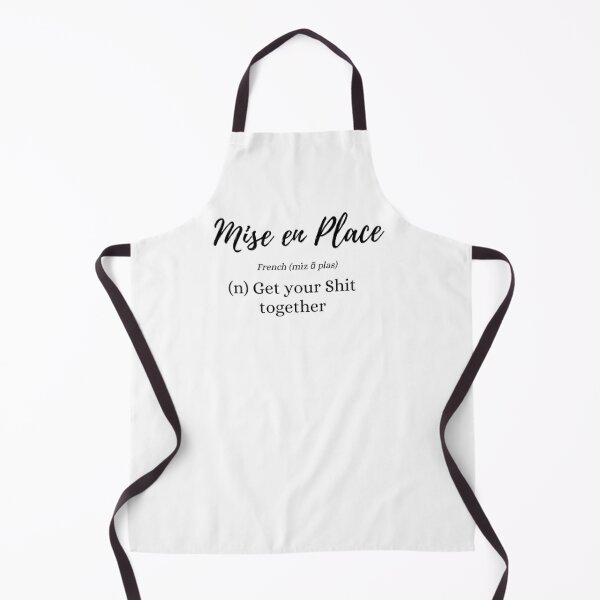This is a detailed product photograph of a white apron with black ties at the neck and shoulders, set against a white background. The apron features a humorous and motivational script in black lettering. At the top, it displays the French phrase "mise-en-place" in a curly, cursive font. Directly beneath, it provides a definition: in italicized text, it says "French," along with the pronunciation of "mise-en-place." Following this, in larger, bold text, the apron humorously defines the term as "Noun, get your shit together," with "get your shit" on one line and "together" on the line below. The apron is laid flat in the photograph, emphasizing its design and text.